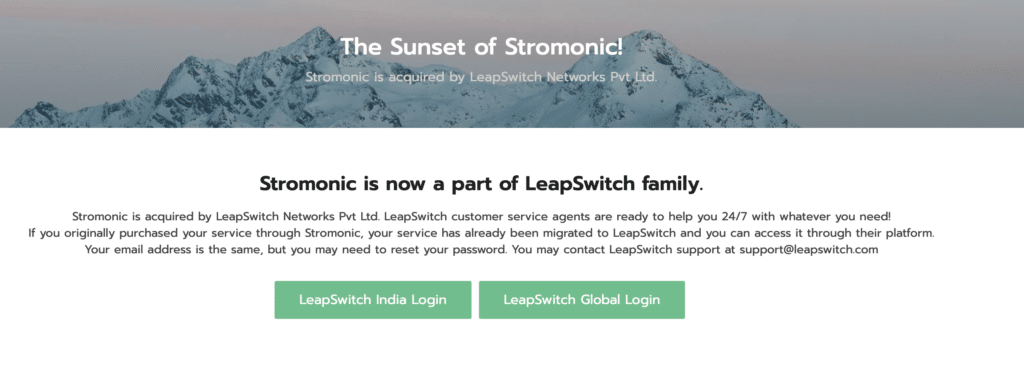The image is a screenshot of a website's front page, prominently displaying an announcement about Stromonic's acquisition by LeapSwitch Networks. The header reads, "The Content of Stromonic," followed by a detailed notice. The notice informs users that Stromonic has been acquired by LeapSwitch Networks, PBT LTD, and is now part of the LeapSwitch family. It emphasizes the continuity of customer service, offering 24x7 support. The notice assures customers that their existing services purchased through Stromonic have been smoothly migrated to the LeapSwitch platform, retaining their email addresses though they may need to reset their passwords. Contact information for LeapSwitch support is provided, directing users to support.leapswitch.com for assistance. Below the announcement, there are two prominent green buttons for logging in: one labeled "LeapSwitch India Login" and the other "LeapSwitch Global Login." The layout is designed to guide both Stromonic's Indian and global customers seamlessly into the LeapSwitch ecosystem.